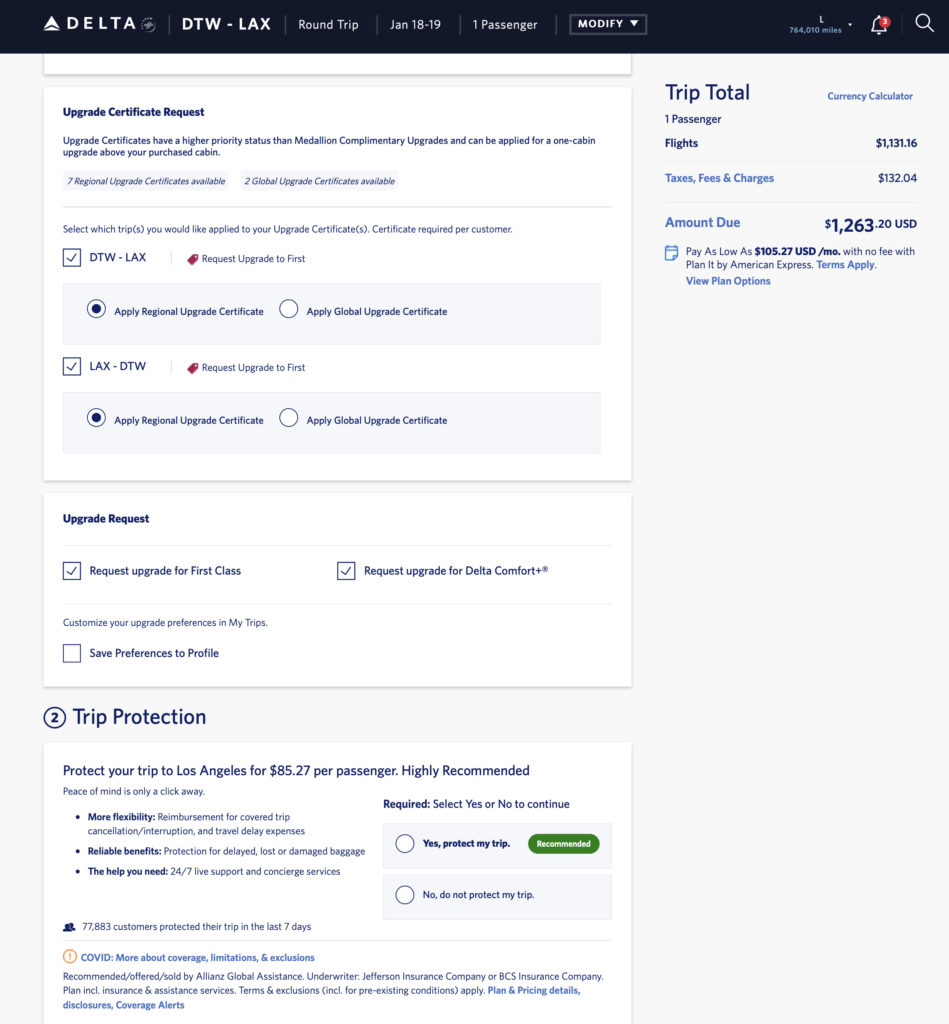Screenshot of a Delta Website page for a flight upgrade request:

In the upper left-hand corner, a blue horizontal bar features the Delta logo in white capital letters, accompanied by a small triangular symbol to its left. Below this bar, the page outlines the flight details, which include a round-trip journey from Detroit Metropolitan Wayne County Airport (DTW) to Los Angeles International Airport (LAX) scheduled for January 18th to 19th for one passenger.

A "Modify" drop-down button is positioned beneath this header. Further down, the main section is titled "Upgrade Certificate Request." Here, the departure flight from DTW to LAX is selected, as well as the return flight from LAX to DTW. Below this, there is an option to "Apply Regional Upgrade Certificate," which is also checked.

The "Upgrade Request" section follows, displaying two checked options: "Request Upgrade to First Class" and "Request Upgrade to Delta Comfort+." The total cost of the trip is listed at $1,263.20.